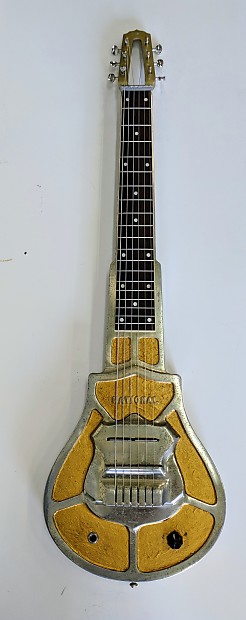The image features a very old electric guitar displayed in an upright position against a light grayish wall. The guitar's body exhibits a distinct mustard-yellow color with a metal faceplate overlaying a wooden base. The body shape resembles a police badge, particularly where the six silver strings converge. The body is sectioned into a mosaic-like pattern with seven distinct yellow segments. Positioned on the lower right corner of the body is a small black dial, while a dedicated input jack is located on the left side. The neck of the guitar is black, leading up to a metallic headstock equipped with tuning pegs. Just below the frets, there is some indecipherable lettering starting with "BAT". A shadow cast on the wall accentuates the instrument, highlighting its vintage aesthetic and the intricate blend of metal and yellow hues.